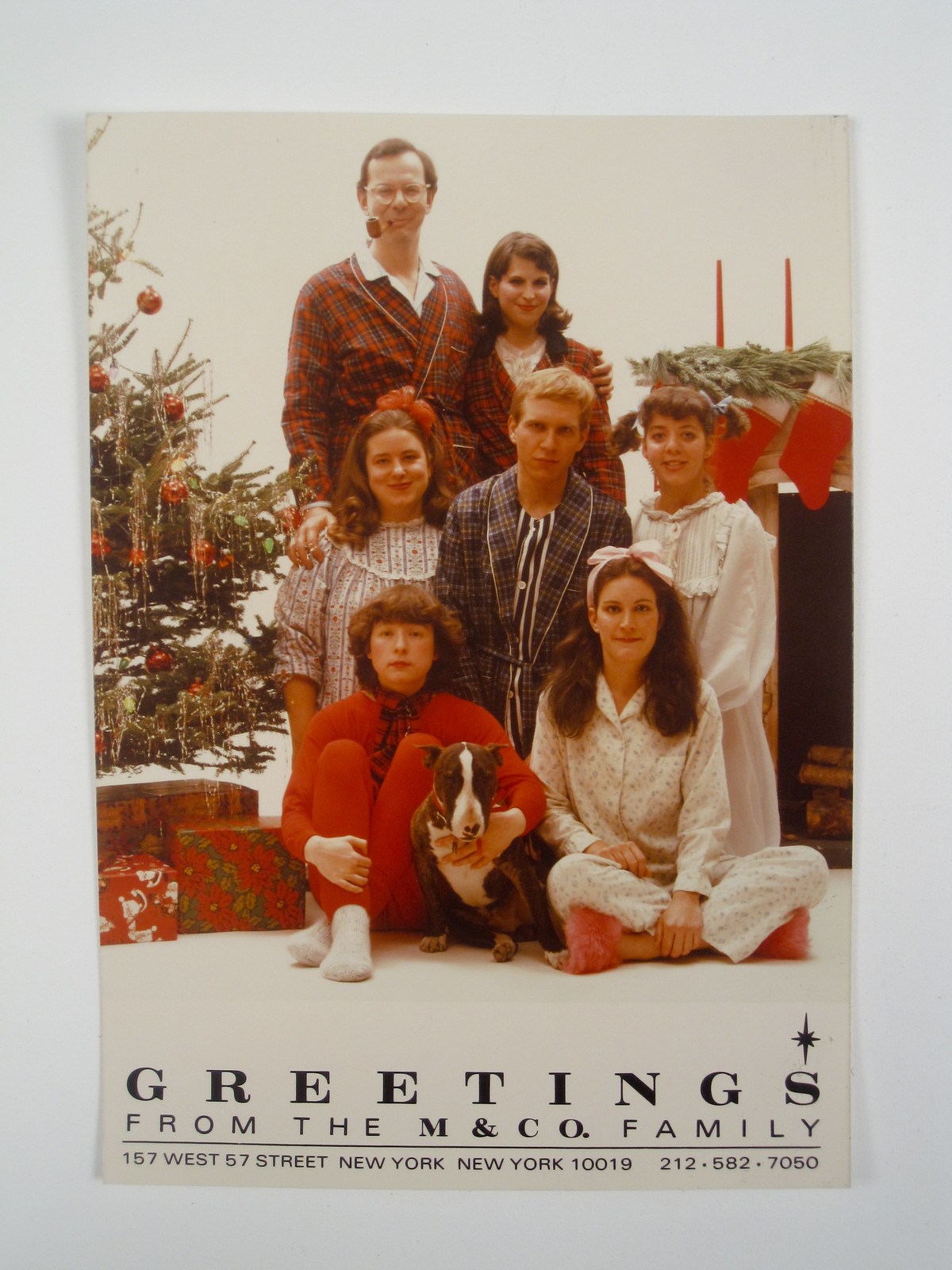The image is a Christmas card featuring a vintage family photograph, likely from the 1970s, depicting a close-knit family of seven along with their dog. At the top of the card is an image showing a family donning Christmas-themed pajamas in red, flannel, and white patterns. Standing in the back are the parents, with the husband wearing glasses and a pipe in his mouth. The middle row includes three children: a daughter, a son, and another daughter. In the bottom row, a son in all red holds a dog, with another daughter kneeling beside him. To the left of the family stands a decorated Christmas tree adorned with presents underneath, and to the right, a fireplace with a mantel decorated with stockings and candles. The bottom of the card bears the text "Greetings from the M&Co Family" in black against a white background, with the address 157 West 57th Street, New York, New York 10019, and the phone number 212-582-7050. The overall setting is a classic, festive Christmas scene centered around family warmth and holiday cheer.